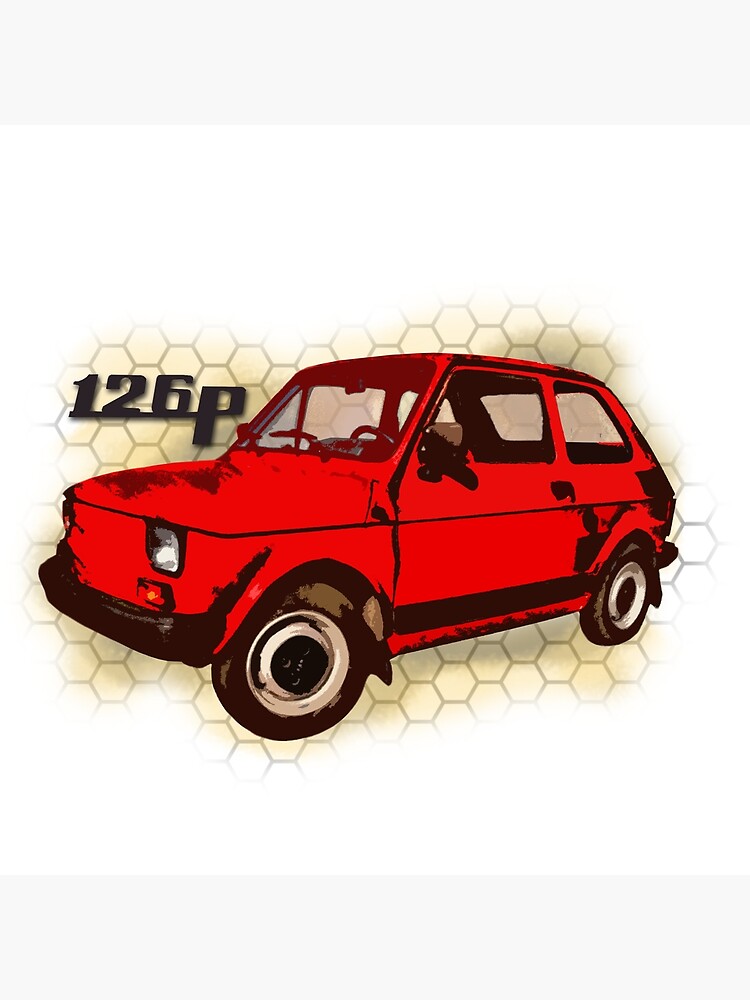This image features a detailed computer-rendered illustration of a bright red, vintage-style, German hatchback, resembling a Volkswagen GTI. The car is viewed from a 3/4 angle, prominently displaying its left front wheel and obscuring the back left tire. The illustration style has been processed to reduce detail, giving it a painted or drawn appearance. Positioned in the center of the image, the car also features the text "126P" just to the left of the windshield. The background is characterized by a distinctive honeycomb pattern with a brown smoky effect, which transitions from a light gray banner at the top to a detailed hexagonal beehive design, adding depth and an intriguing visual texture to the composition.